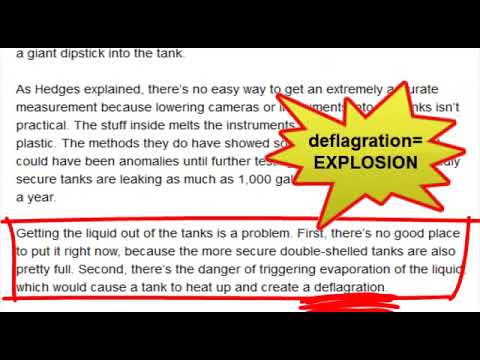The image features a white background flanked by black banners at the top and bottom. Centrally located is detailed black text discussing an engineering issue regarding liquid removal from tanks. The lower portion of the text is highlighted by a red box, within which it explains the dilemma: the more secure double-shelled tanks are nearly full, and removing the liquid risks triggering evaporation, leading to tank heating and potential deflagration. Above this, a large jagged text bubble, bordered in red with a yellow center, emphatically states "DEFLAGRATION = EXPLOSION" in bold black letters, underscoring the significant danger involved.